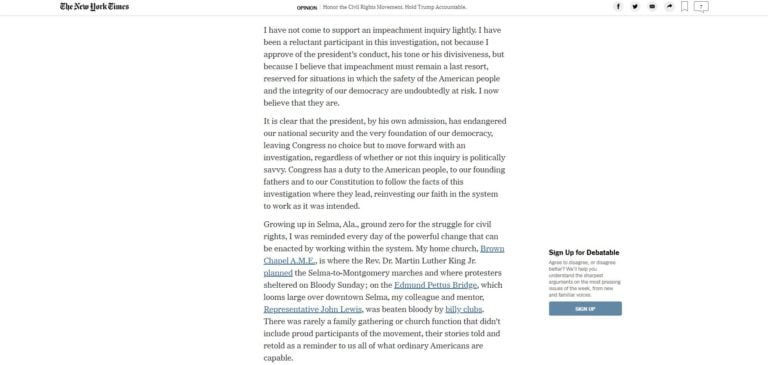"The article featured is from The New York Times, with the publication's banner clearly displayed at the top left under the 'Opinion' section. The headline appears to emphasize accountability for former President Trump and the protection of the civil rights movement. The author discusses their initial reluctance to support an impeachment inquiry into Trump's conduct. Despite not approving of his behavior or rhetoric, they highlight the importance of impeachment as a last resort, necessary only when the safety of the American people and the integrity of democracy are at risk. The article argues that President Trump, through his own actions, has jeopardized national security and democracy, leaving Congress with no alternative but to proceed with an investigation. The piece underscores Congress's responsibility to the American people, the Founding Fathers, and the Constitution to pursue the investigation impartially. The author recounts experiences growing up in Selma, Alabama, and concludes with a call to participate in a debate. The opinion piece reflects a deep concern for the nation's future amidst the political turmoil.”